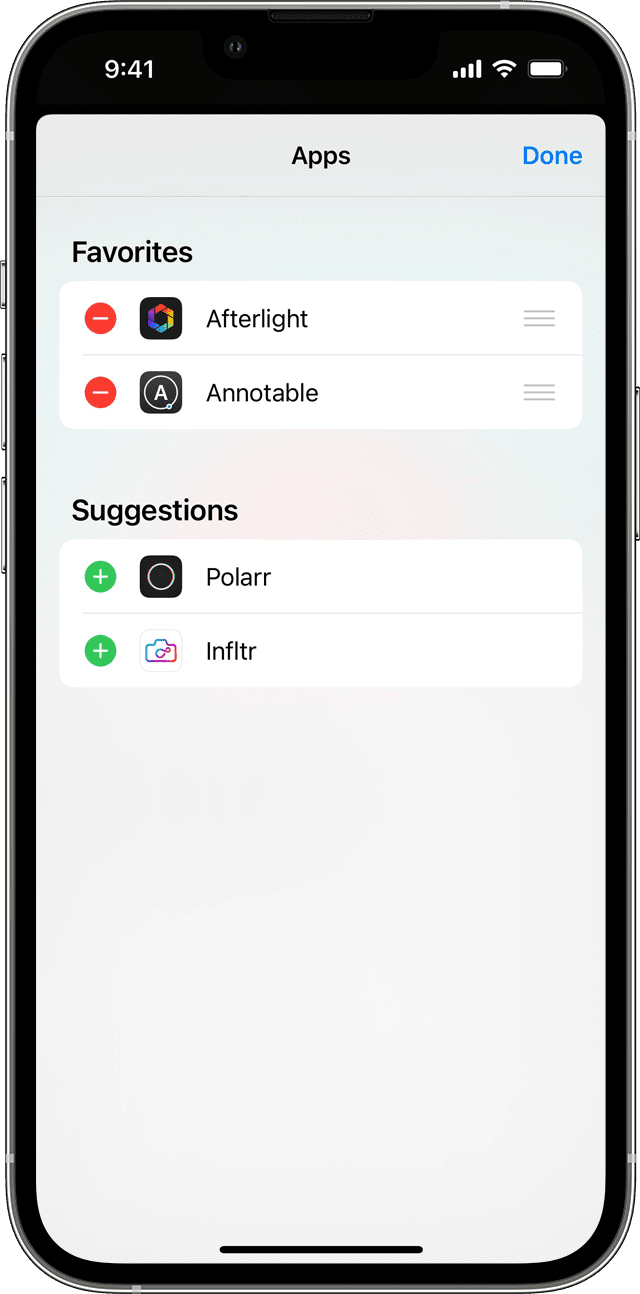In this image, a sleek black cell phone stands vertically against a solid white background. The device features three silver buttons on its left side—two of them longer and positioned below a smaller, top button. On the right side, there is a single silver button. The phone's screen prominently displays a white background with the word "Apps" centered in black text. Above this, a black bar shows the time "9:41" in white text, along with four white bars indicating full reception, an active Wi-Fi symbol, and a fully charged battery icon located in the upper right corner. Below "Apps," on a very light gray background, is the word "Favorites" in black text. Directly underneath "Favorites" are two white lines displaying app names: the first one reads "Afterlight," accompanied by a black square icon to its left, and the second line reads "Notable," featuring a black square icon with a white letter "A" inside.